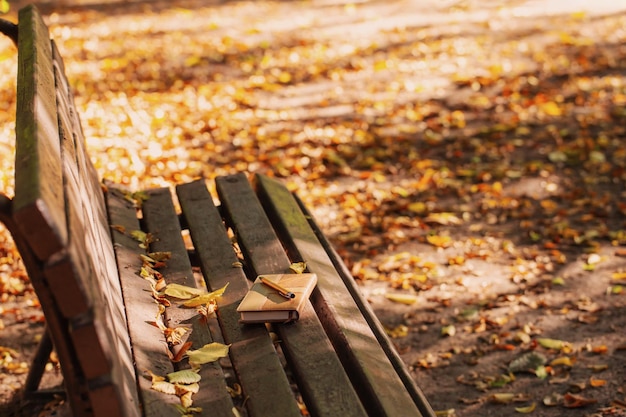A beautifully composed photograph captures an outdoor wooden park bench, viewed from the side such that its seat points towards the upper left corner of the image. The bench, constructed with dark brown wooden slats and reinforced with metal legs and back, sits on a light gray dirt ground scattered with vibrant fall leaves in shades of yellow, orange, and occasional greens. The background is blurred, emphasizing the bench and its contents, while hinting at the fall season with partially visible leaves. On the bench seat, a light brown journal lies closed with its spine facing outward. Atop the journal rests a pencil, specifically a gold pen with a clip, oriented towards the back of the bench. The simplicity and autumnal atmosphere of the scene evoke a sense of calm and solitude. There are no people in the image, only the bench, leaves, book, and pen providing a snapshot of a quiet moment in nature.